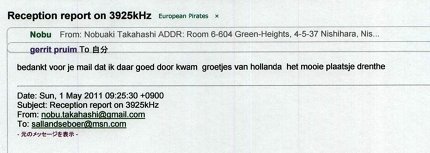This image depicts a cropped email slip with a white background and predominantly black text, though some portions are green and dark blue. At the top, the text reads "Reception Report on 3925KHZ European Pirates". Beside it in green, it says, "From Nobuaki Takahashi." Below, there’s an address: "Room 6-604, Green Heights, 4-5-37 Nishihara." Following these details, there is a block of text in a foreign language, possibly Japanese. Further down, the email indicates it was sent on "Sunday, May 1st, 2011, at 09:25". A recipient email address and other foreign text follow, although these parts are not clearly understood.